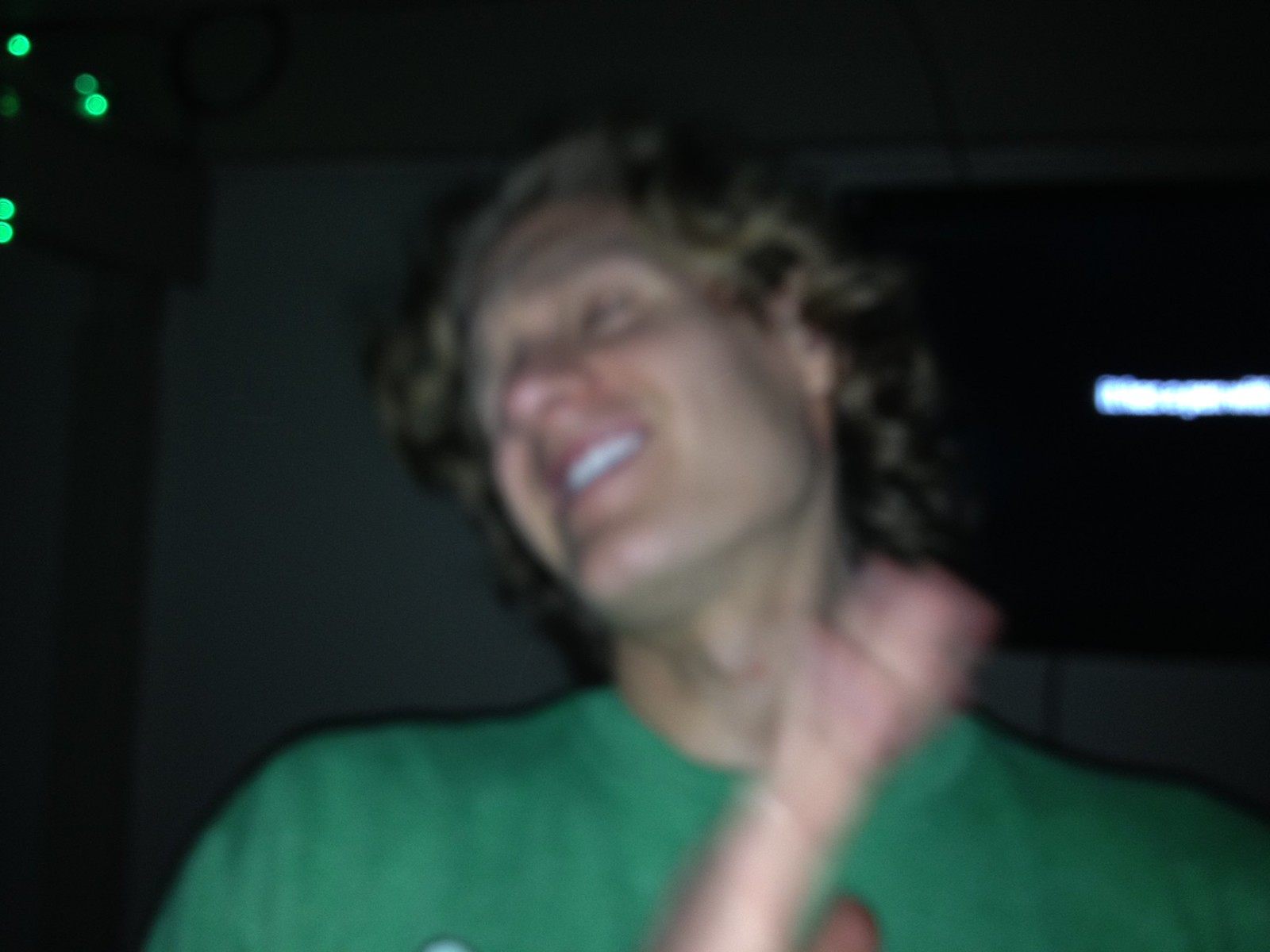The image depicts a nighttime outdoor scene, captured with a flash camera. The central focus is on a person who appears blurry due to long exposure and slight camera movement. The person is well-lit by the flash and is seemingly wearing a green T-shirt. Their hand extends from the lower border of the frame at a sharp angle, likely pointing upwards. Despite the blurriness, the individual's head is tilted to the left, and they display a bright white smile. They have medium-length shaggy brown hair and are clean-shaven.

The background is predominantly black, indicating the dark surroundings. On the right edge, midway up the image, there's an overexposed white bar that could be a set of car headlights or a store sign. In the upper left corner, a collection of blurred green light dots is visible, potentially streetlights or another distant light source. Despite the blurriness, these dots appear unusually distinct and numerous, adding a mysterious element to the scene.